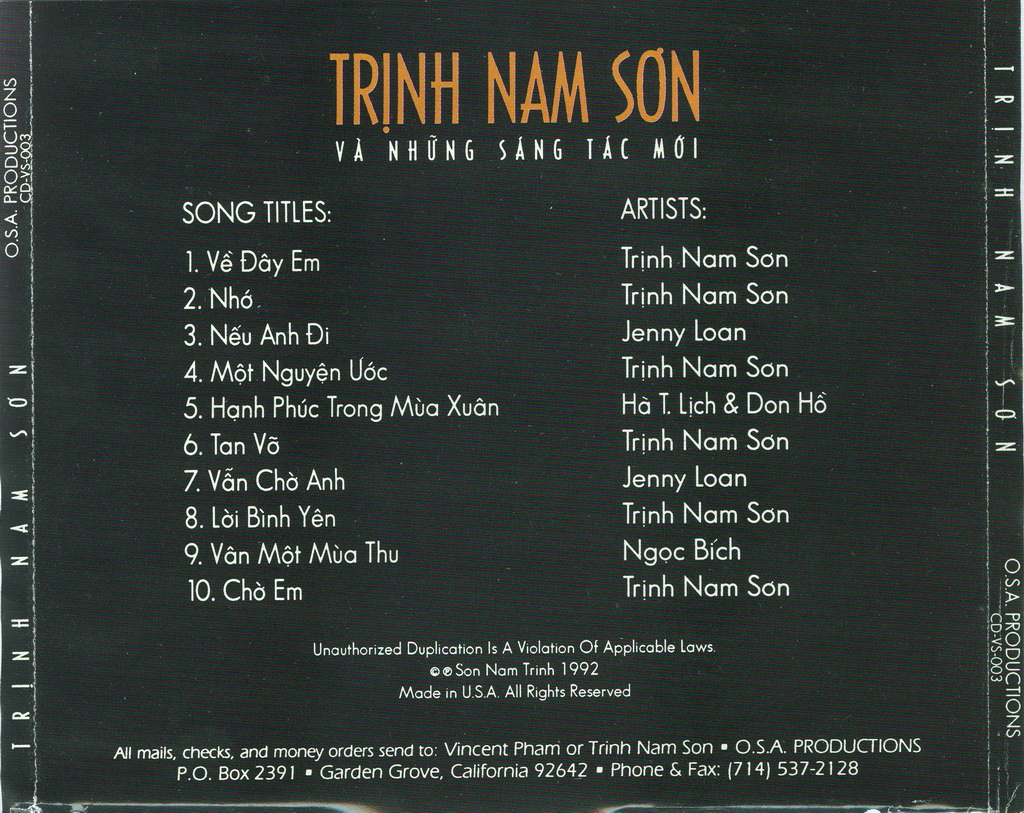This is the cover of a black-and-white music CD compilation titled "Trin Nam Son" by O.S.A. Productions. The only colored text on the cover, in orange capital letters, reads "TRIN NAM SON" at the top center. Below that, in small white lettering, it says "Vahung Sang Tak Moi," which might be in an Asian language. The cover is designed with two columns; the left column lists the song titles, and the right column lists the artists. 

There are ten song titles in total, and five different artists featured. Most of the songs, including the first two, the fourth, the sixth, and the last, are by Trin Nam Son, who is emphasized throughout the cover. Other contributing artists include Jenny Loan (third and seventh songs), Ha Thi Leach and Don Ho (fifth song), and Ngoc Bich (ninth song).

The bottom of the cover includes a note against unauthorized duplication, along with copyright information: "Copyright SON NAM TRIN, 1992, made in USA, all rights reserved." It also provides contact details for purchasing the CD, with instructions to send mail checks or money orders to Vincent Pham or Trin Nam Son at O.S.A Productions, located at a P.O. Box in Garden Grove, California, along with the provided phone and fax number.

Additionally, the name "TRIN NAM SON" is repeated vertically along the left and right borders of the cover, reinforcing the artist's prominence. The CD number "V-S-OO-3" is also printed by O.S.A. Productions, indicating its catalog reference.